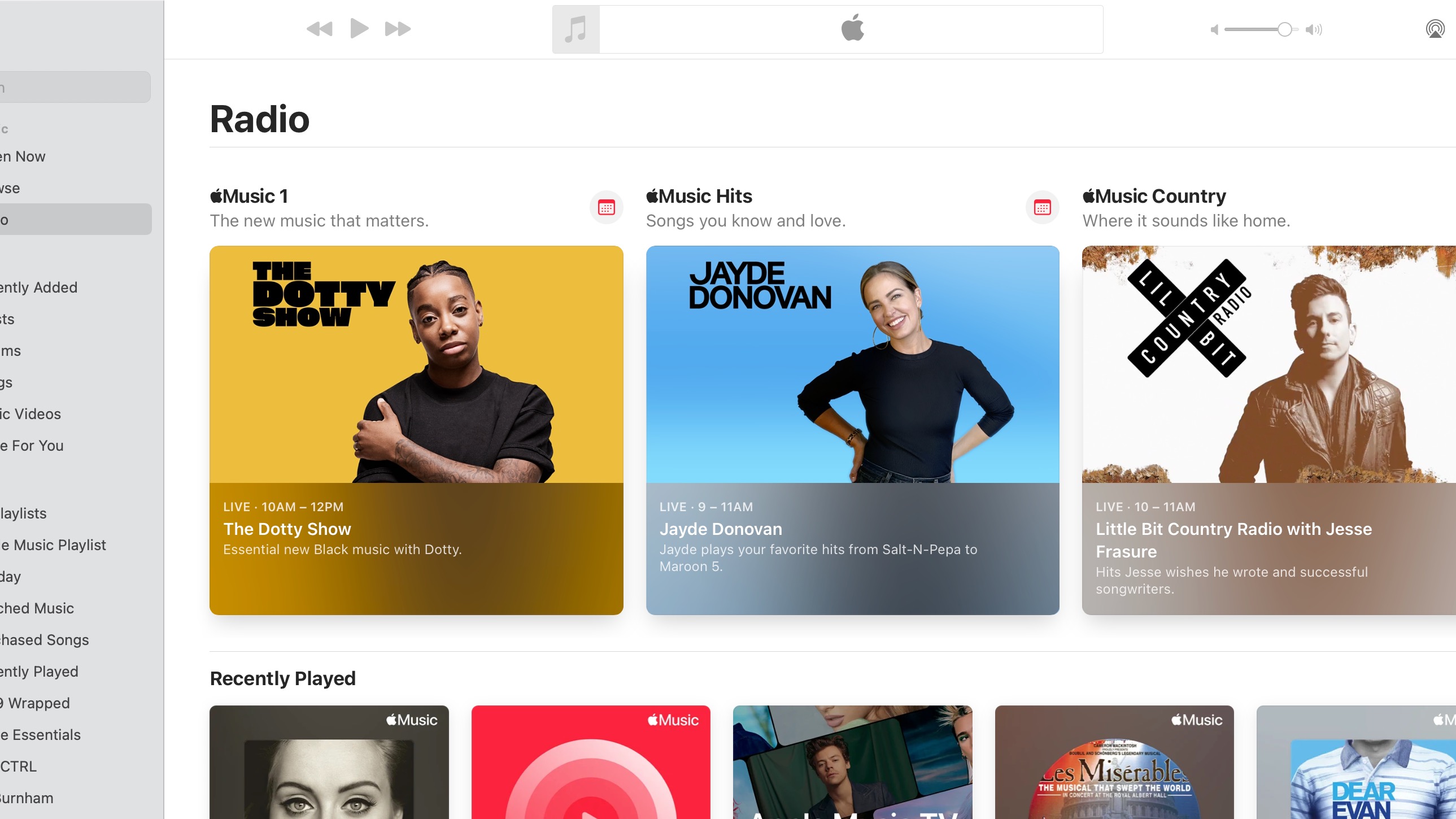The screenshot appears to show the interface of iTunes, identifiable by the Apple and iTunes logos in the top middle portion. On the left-hand side, there's a light gray division with text that's largely unidentifiable, though some apparent snippets include phrases like "frequently added," "videos for you," "playlists," "music playlists," "search music," "chased songs," "currently played," "wrapped," "essentials," and "CTRL." 

The predominant part of the screenshot features a white background. Below the Apple and iTunes logos, there are basic playback control buttons: a rewind button, a play button, and a forward button. Moving further down, there's a heading labeled "radio," under which several content options are listed.

Two main shows are highlighted:

1. "The Dottie Show" - Live from 10 a.m. to 12 p.m., hosted by Dottie. The show is described as "essential new black music with Dottie." Dottie is depicted as an African American woman with cornrows, posing with her right hand clutching her left shoulder.

2. "JAYDE" - Another show running live from 9 to 11 a.m., hosted by J.D. Donovan. It mentions J.D. playing fan-favorite hits ranging from Salt-N-Pepa to Maroon 5. Jayde is shown as a female figure with both arms on her hips, wearing a black long-sleeve shirt without a collar.

Overall, the screenshot provides a quick look into iTunes' radio offerings, showcasing two specific music programs with detailed descriptions and host images.